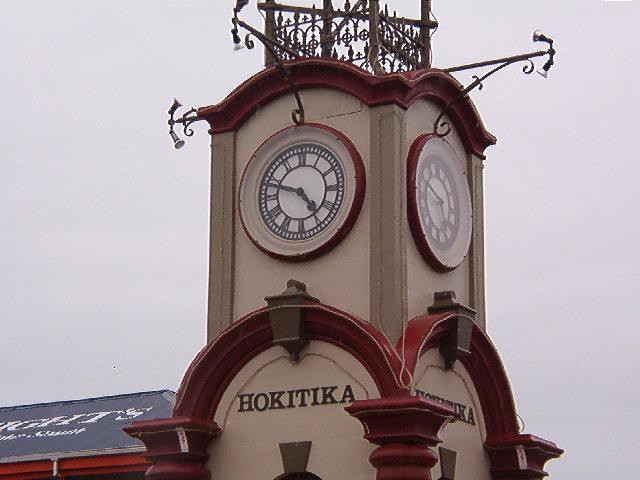The colour photograph features the top section of a muted beige clock tower, adorned with an arched brownish-red top. This section is fenced with small decorative iron pieces, possibly wind vanes. The tower prominently displays two large, round clocks—one facing the front and another on the right—both of which are encircled by a red outline with a pale tan inner ring that complements the tower's color. The clock faces are white with black Roman numerals and feature black hands, set to approximately 4:50. Each clock is illuminated by dual metal arms extending outward with light bulbs. Below the clocks, the structure widens with another red arched border that contains the text "HOKITIKA" in brown letters. The background is a grey sky, enhancing the muted tones of the scene. In the lower left corner, a slanted grey roof with red trim is visible, bearing some barely legible white text that includes the letters "NGHTS."